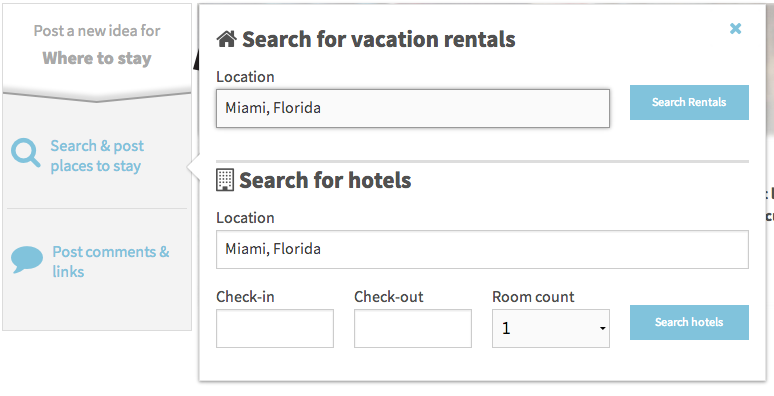This rectangular image appears to be a screenshot of search results from a vacation rental and hotel booking website. Dominating the center of the image is a large white window with a dark gray outline. 

On the left side of the window, there is a house icon followed by the text "Search for vacation rentals" in dark gray. Beneath this, the word "Location" is displayed with a text bar below it that indicates "Miami, Florida." This text bar is outlined in either black or dark gray. Adjacent to the text bar on the right, a small rectangular button in blue with white writing reads "Search results."

Below this section, there is another heading in dark gray that reads "Search for hotels." Again, "Location" is displayed with a text bar underneath that, also reading "Miami, Florida." Further down, there are three options labeled "Check-in," "Check-out," and "Room count." Each of these options has an associated text field or drop-down menu; specifically, "Check-in" and "Check-out" have text fields under them, and "Room count" has a drop-down menu showing "1." To the right of these fields, there is another rectangular button with a light blue background and white text that reads "Search hotels."

Additionally, on the far left side of the image, a menu with three rectangular options is visible. These options are titled "Post a new idea," "Where to stay, search and post places to stay," and "Post comments and links."

Overall, this detailed layout provides a comprehensive interface for users to search for vacation rentals and hotel accommodations in Miami, Florida.